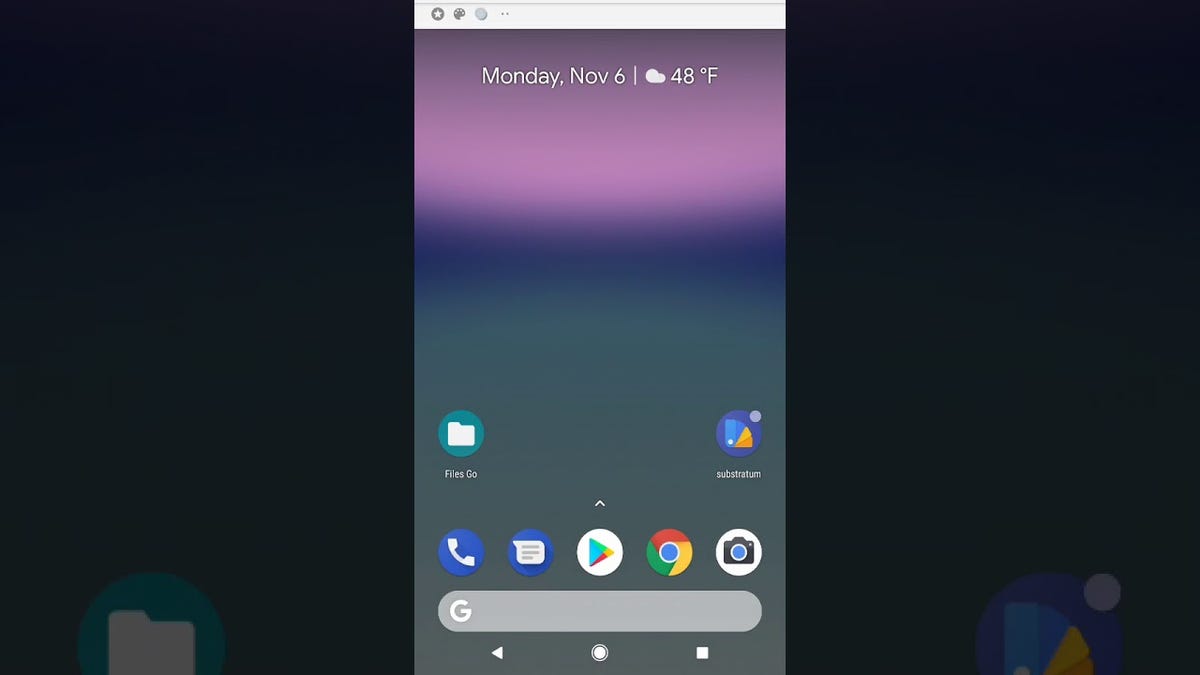This image captures the screen of a cell phone with notable details in the background as well. The focal point highlights two apps: 'Files Go' on the left and 'Substratum' on the right, prominently displayed on the phone screen. The background features a black rectangle with a few items, giving a zoomed-in perspective.

The upper section of the cell phone screen is predominantly white. As you move down, the background transitions through a gradient, starting with a purplish hue, then shading into navy blue, and finally a gray hue at the bottom. Below the main apps, in a smaller size, 'Files Go' and 'Substratum' reappear. Further down is a row of app icons, including a phone icon, a speech box icon, Google Play, Google Chrome, and a camera icon. At the very bottom, there's a search bar with a 'G' inside it, indicating Google's signature search functionality.